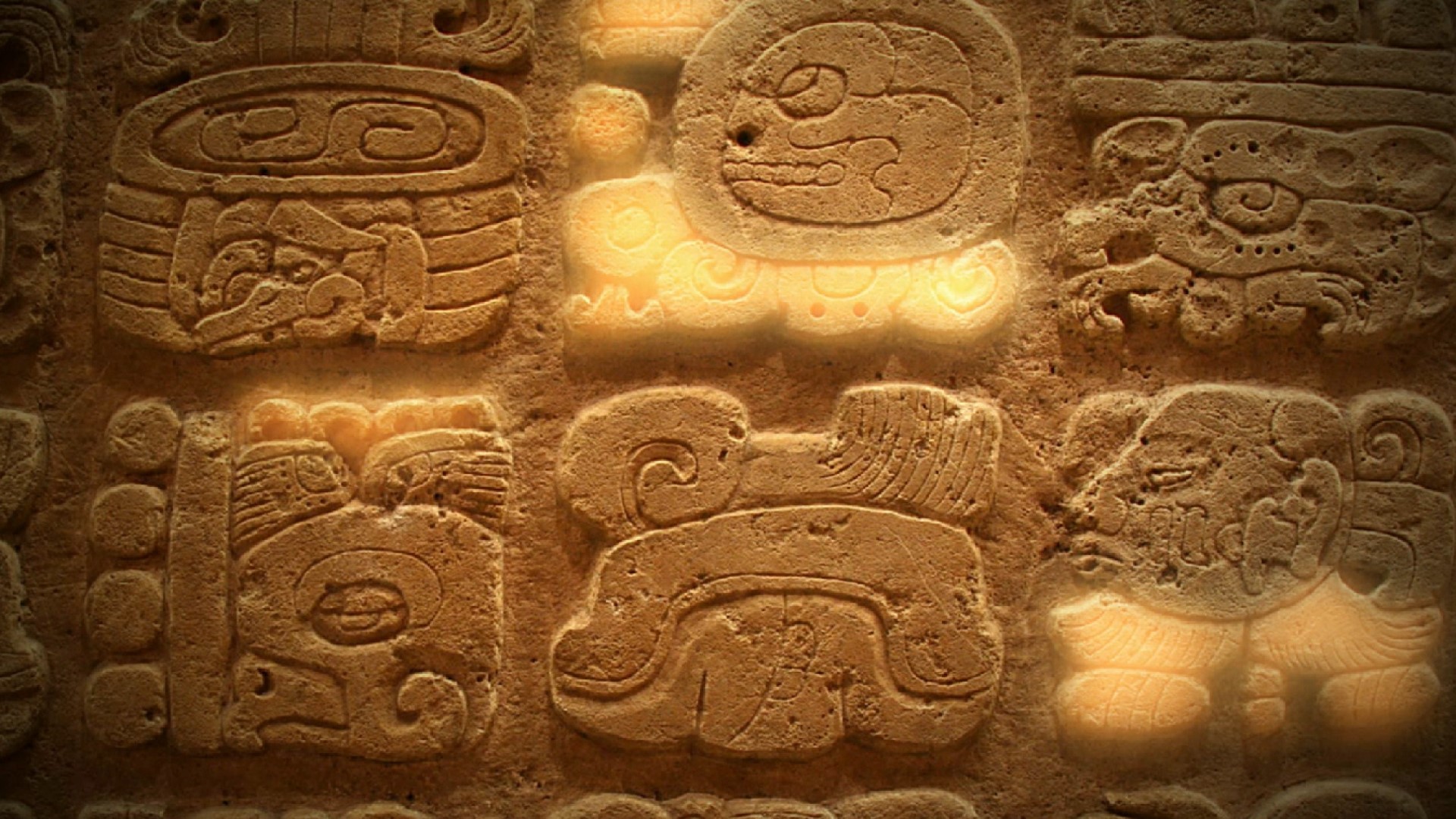The image depicts a beige sandstone-esque wall, likely part of a tunnel or cave, intricately etched with detailed carvings that give off an ancient, hieroglyphic-like vibe, though they are more elaborate. The carvings are spread across six distinct areas on the wall. 

In the upper left, there is a circular design resembling a vase or pot with three vertical stripes and a swirled pattern at the top. The upper middle section features a face with an angered expression looking to the left, surrounded by a brighter wave-like pattern beneath it. The upper right contains a hard-to-identify etching, possibly resembling a porous rock wall. 

In the bottom left section, there are four clearly carved circles, a vertical line, and an eyeball complete with a detailed iris and a strange 'L' shape emerging from it. The central part of the wall presents an image reminiscent of a crashing wave over a beachhead. Finally, the bottom right showcases a stoic-looking man's face with a prominently carved ear, accompanied by faintly glowing, feather-like lines beneath.

Throughout the image, various shapes, faces, circles, ovals, and swirls are illuminated by light hitting specific parts of the carvings, enhancing their visibility and adding to the mysterious, almost narrative quality of the etchings.